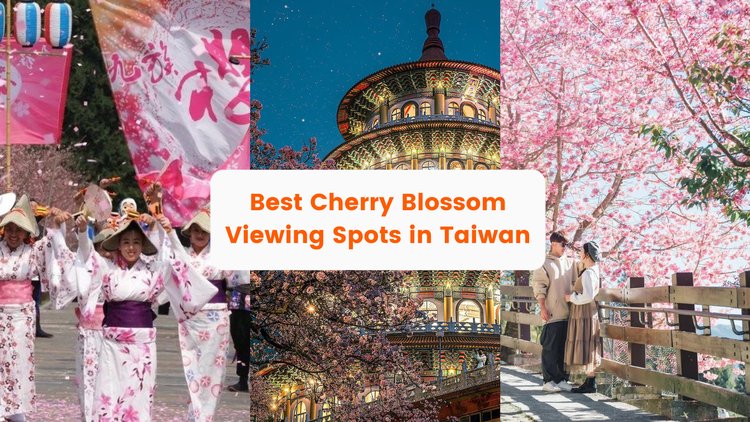This image is a composite of three photographs showcasing the best cherry blossom viewing spots in Taiwan, with a white text box in the middle adorned with orange letters proclaiming "Best Cherry Blossom Viewing Spots in Taiwan."

On the left, a group of Japanese women dressed in traditional attire, featuring white and pink dresses with purple and pink belts, are posing against a backdrop of cherry blossom petals and a flag in pastel colors. 

The center photo depicts a grand, circular Taiwanese building illuminated at night, surrounded by the delicate pink blooms of a cherry blossom tree against a vibrant blue sky.

To the right, a serene scene unfolds with a man and a woman standing next to a wooden fence under a massive cherry blossom tree. The sunlight casts intricate shadows from the fence onto the ground, highlighting the couple's neutral clothing and making the pink blossoms behind them stand out prominently.

Together, these images encapsulate the breathtaking beauty of cherry blossom season in Taiwan.